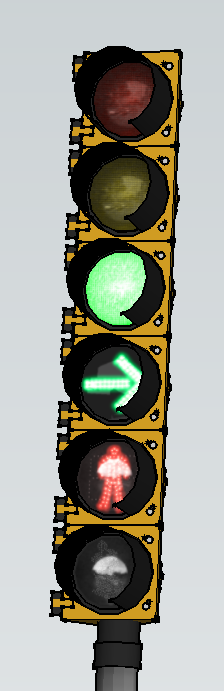The image depicts a detailed drawing or painting of a traffic light pole showcasing a unique configuration of six different signals. Starting from the top, the lights are arranged as follows: a traditional red light, an amber light, a green light, a green right-pointing arrow, a red "no walking" person, and an unlit bottom light presumed to be a pedestrian symbol. The traffic light apparatus is mounted on a gray pole, with the signal housing presented in a vibrant yellow hue and the circular light housings in contrasting black. The illuminated lights in the scene include the green light, the green arrow, and the red "no walking" person. The entire scene is set against a minimalist background in shades of light grey, emphasizing the traffic signal's colorful details and elongated, rectangular format.